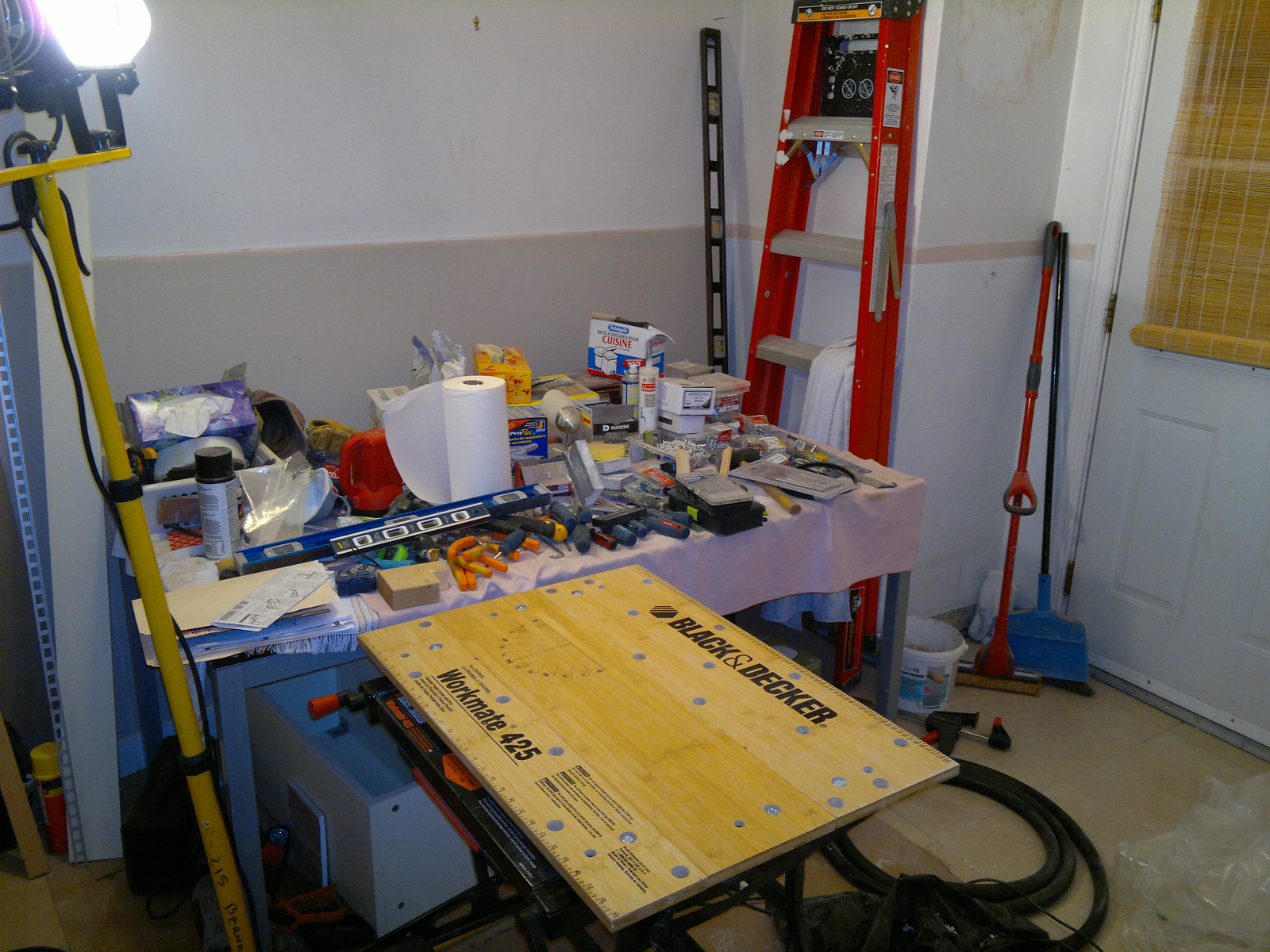A neatly organized table is set up against a wall in what appears to be a utility room. The rectangular table, draped in a pristine white linen cloth, has a metallic frame. Resting upon it is a collection of various tools and supplies. From left to right, there is a row of neatly arranged paper towel rolls, a selection of screwdrivers, spanners, tubes of caulk, and several spray cans. Amidst these items, a bright yellow box of facial tissues stands out. To the right of the table, a white door is visible, leaning against which are a broom with a black and blue handle and a mop with a red stick. Nestled between the wall and the table is a red ladder, adding a splash of color to the utilitarian setting.